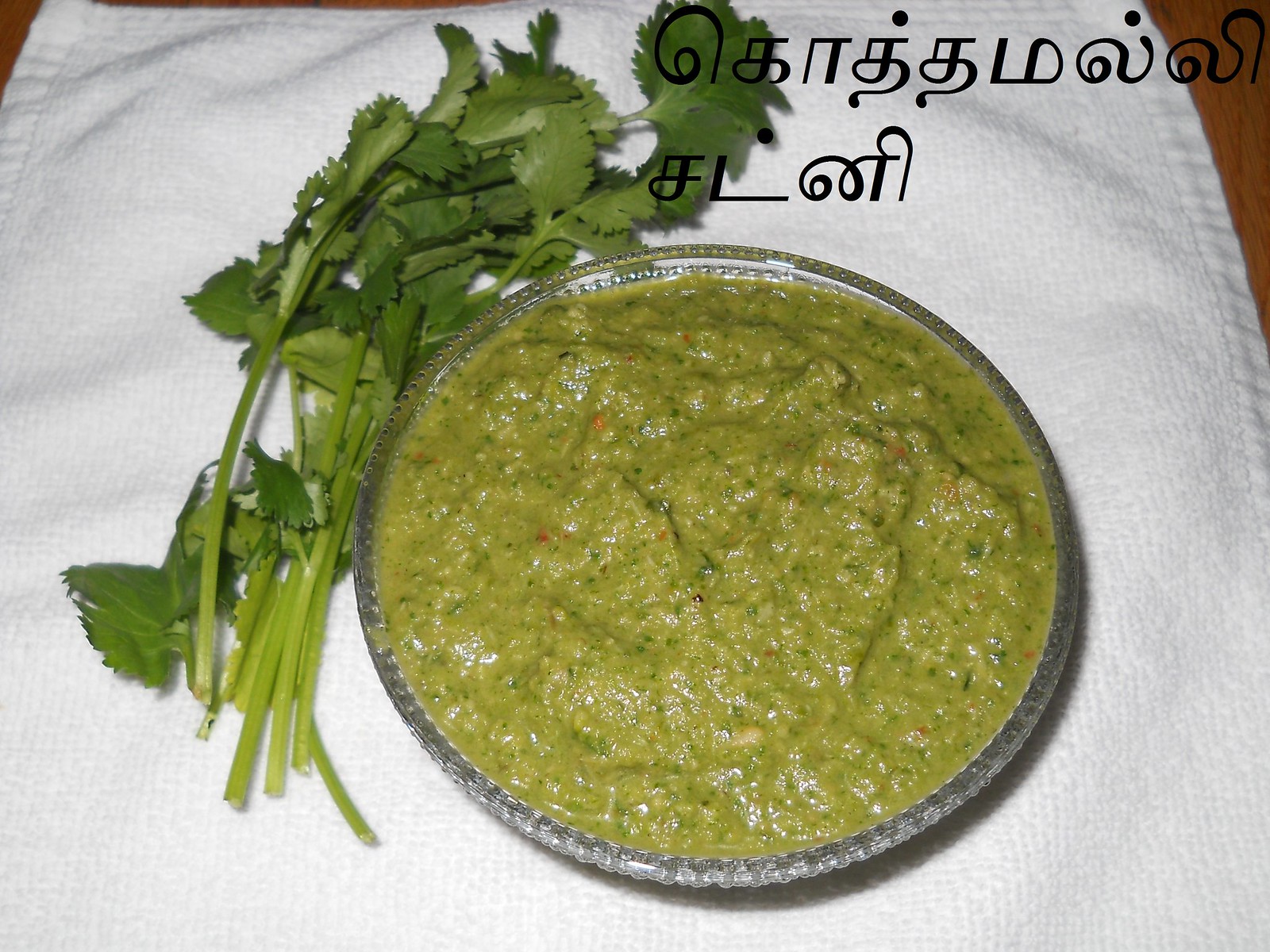This close-up image features a circular glass bowl with a beveled edge, containing a vibrant green paste that resembles guacamole. The paste is richly textured with tiny pieces of chopped cilantro, and is speckled with orange and red flecks, likely red pepper flakes or another seasoning. The bowl sits atop a white towel, which itself rests on a brown wooden table, faintly visible at the upper left and right corners of the image. To the left of the bowl, there are several sprigs of cilantro, approximately seven or eight in total. In the upper right-hand corner of the image, there are black letters in an unfamiliar language. The overall presentation suggests a flavorful dip, garnished and seasoned to enhance its appearance and taste.